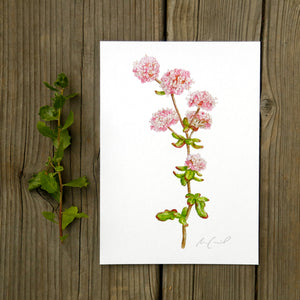This is a detailed photograph of a painting of flowers displayed on an unfinished wooden plank background, resembling a picnic table. The painting, created on a white piece of paper, features a tall stalk with six large, bushy flowers, possibly peonies, due to their thick foliage. The flowers, depicted in shades of pink, white, and red, are arranged with two at the very top, three just below that, and one halfway up the stalk. Green leaves adorn the bottom of the stem, matching a single branch with similar leaves positioned to the left of the painting. The wooden background is made up of lined planks with a thick line noticeable between two central boards. The painting is signed in the bottom right corner, although the signature is unreadable.